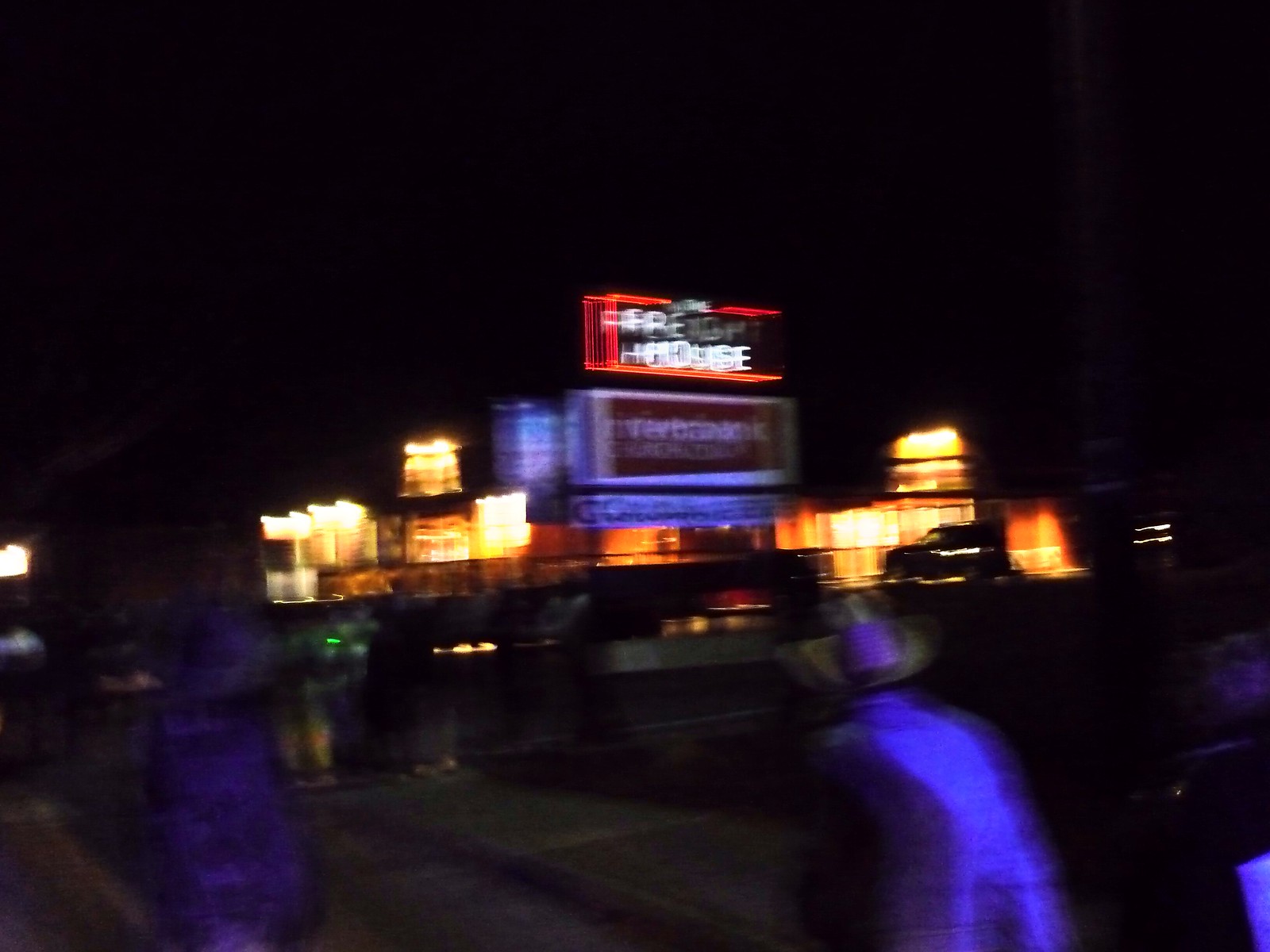A blurred nighttime photograph captures a scene from a boardwalk. In the lower part of the image, two figures are visible with their backs turned to the camera. The person on the right is wearing a purplish hat. In the background, a city skyline is faintly discernible, with buildings illuminated against the expansive, dark sky that dominates the majority of the frame.